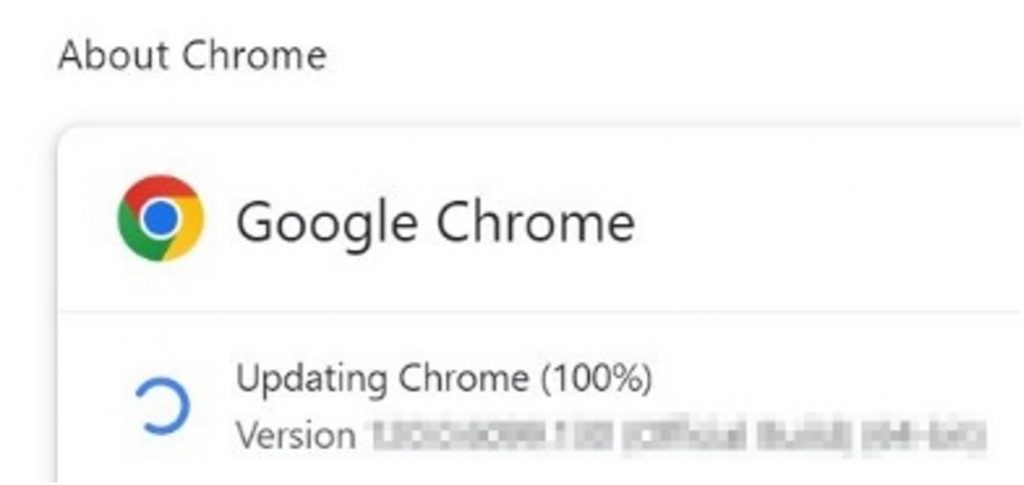The image is a small screenshot focusing on the "About Chrome" section of the Google Chrome browser. At the top, there is text that reads "About Chrome". Below this, the iconic Google Chrome logo is prominently displayed. The logo is a circular emblem divided into three colored sections: red, yellow, and green, with a blue circle in the center. Adjacent to the logo, the text "Google Chrome" is clearly visible. Beneath this, a blue icon resembling a backward 'C' is present, alongside text indicating "Updating Chrome 100%". Further down, there is a line that begins with "Version," but the specific version information has been intentionally blurred for privacy reasons. The image is devoid of any additional elements such as people, animals, plants, buildings, signs, mechanical objects, or vehicles. Its sole focus is the update status of the Google Chrome browser.